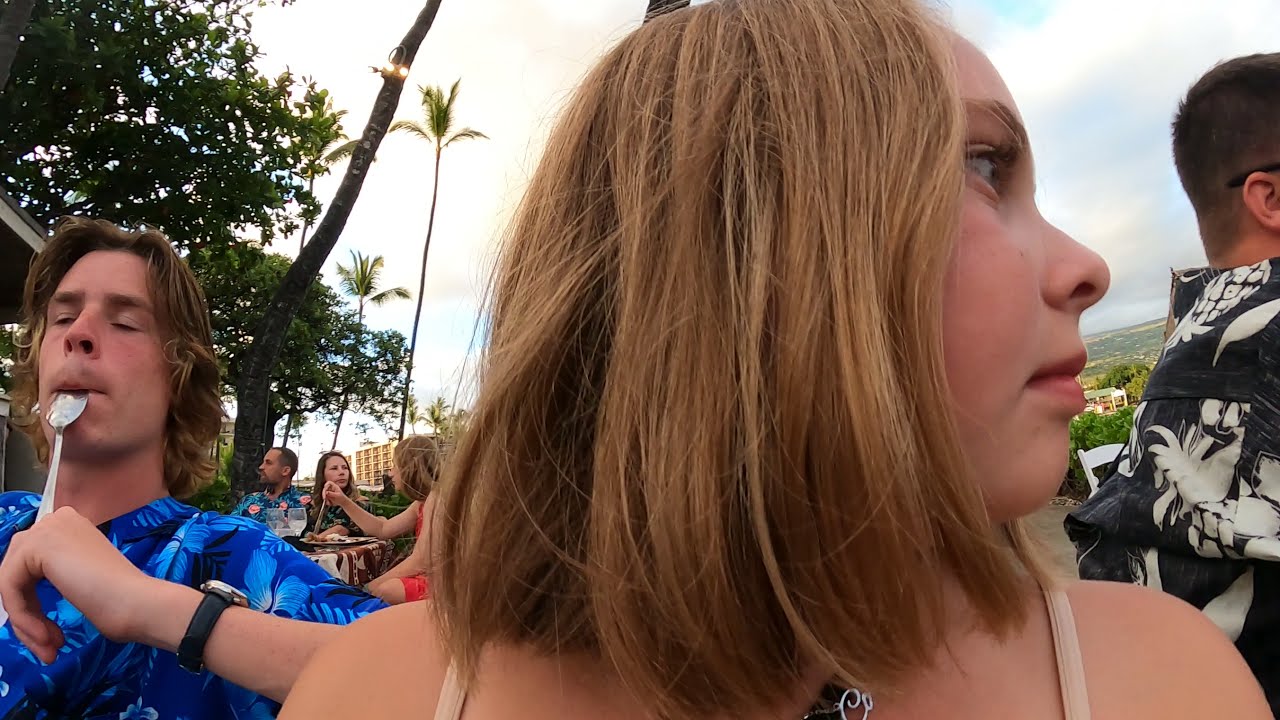In an outdoor eating area under a clear blue sky, a young girl with strawberry blonde hair is depicted in profile, facing to her left. She's wearing a spaghetti strap top that reveals her shoulders. To her immediate left, a man with long light brown hair, a mustache, and a blue two-tone shirt has a spoon hanging from his mouth, his eyes closed, and he's wearing a black wristwatch. Behind her, farther in the background to her right, are two women and a man seated at a table, engaged in eating. The man at the table wears a flowered shirt. On her direct right, partially visible, is a man wearing a black shirt with white print. The scene is set against a backdrop featuring trees, including a palm tree, and in the distance, a tall building that appears to be a hotel.